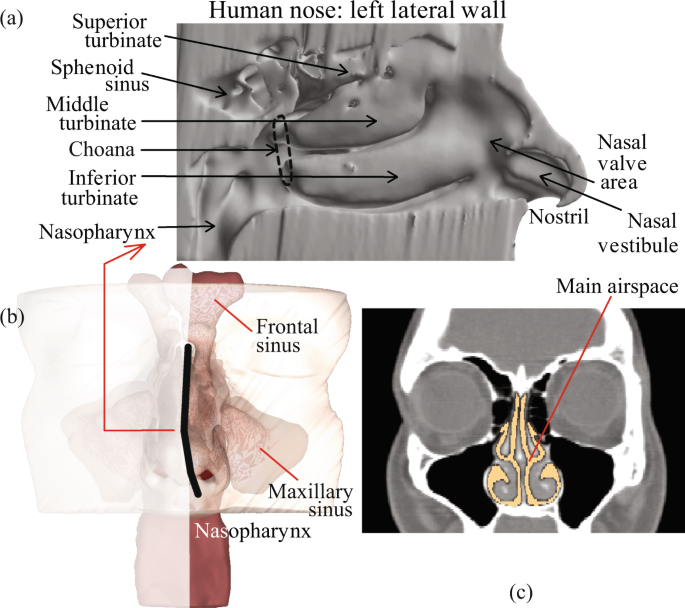The image consists of three detailed medical illustrations of the human nose, each highlighting different perspectives and anatomical features. 

The top illustration, labeled as Image A, provides a comprehensive view of the left lateral wall of the human nose. This side view intricately labels various parts, including the superior turbinate, sphenoid sinus, middle turbinate, choana, inferior turbinate, nasopharynx, nasal valve area, nostril, and nasal vestibule.

Image B, situated beneath Image A, offers a 3D-like depiction of the frontal section of the nasal area. Key features such as the frontal sinus, maxillary sinus, and nasopharynx are clearly labeled and color-coded in red and white for better differentiation.

Lastly, Image C presents an X-ray view of the human nose from the front, emphasizing the main airspace. This image highlights the primary pathway through which air enters the nasal cavity.

Together, these illustrations provide a thorough and multi-faceted anatomical study of the human nose, showcasing various internal structures and sinuses from different perspectives.